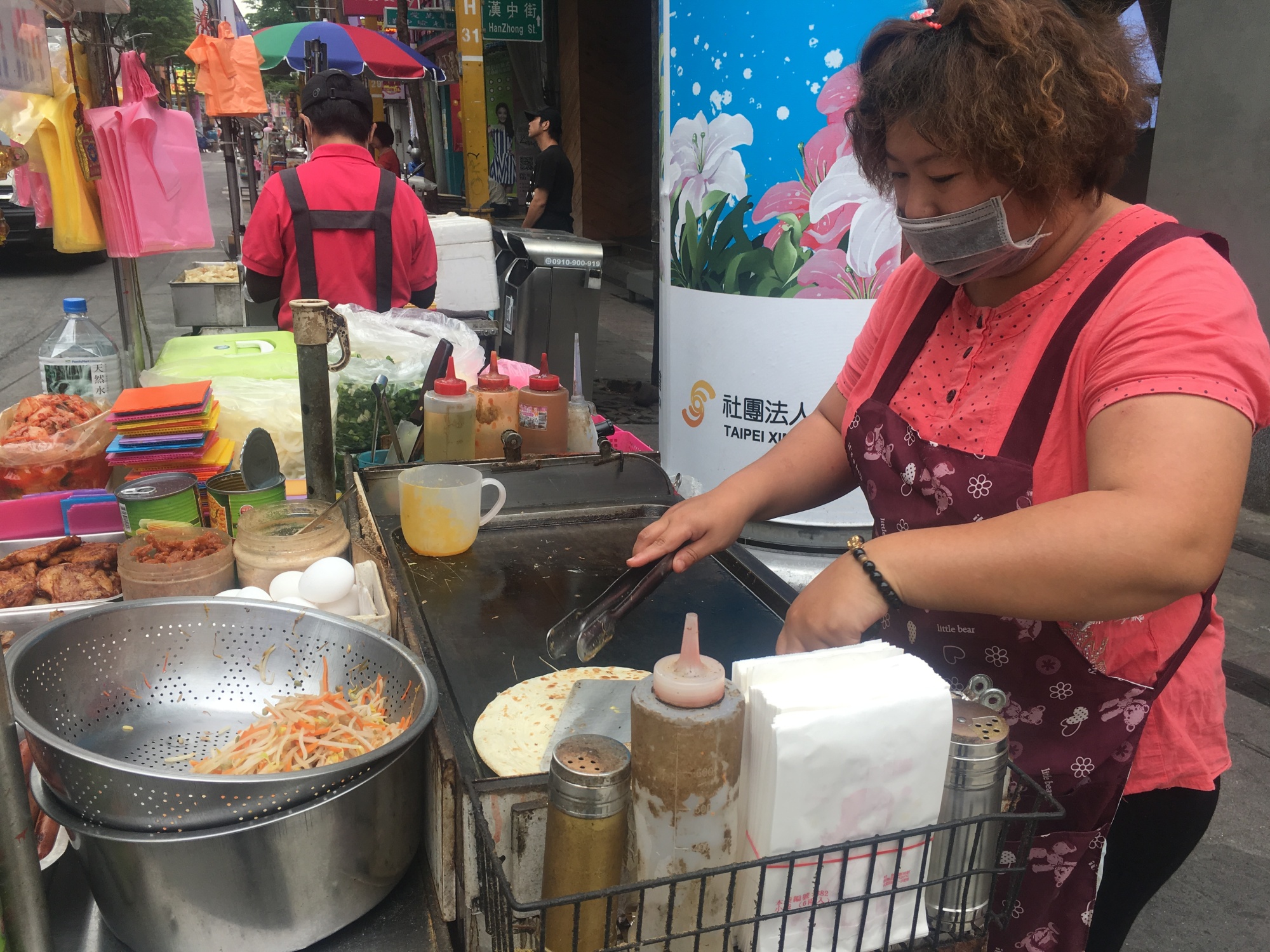In this bustling street scene set in Taipei, an Asian woman stands at a mobile street vendor cart, framed by a vibrant backdrop featuring a white poster with pink and white flowers. The woman, donned in a pink shirt and a burgundy apron adorned with flowers, wears a face mask as she diligently prepares a meal. Her medium-length brown hair peeks out from behind the mask as she works over a silver cooktop. A tortilla sizzles on the griddle while she holds cooking utensils in her hands. To her right, a black basket holds various spices and condiments in squeeze tubes, alongside paper bags. In front of her, an array of food items, including chopped vegetables, meats, and boiled eggs, are neatly arranged in containers and strainers. Serviettes and other cooking essentials dot the scene. On the left side of the frame, a man dressed similarly in a red apron stands with his back to the camera, contributing to the lively atmosphere typical of street food markets. The background reveals a busy street lined with more vendors, adding layers of color and activity to the image.